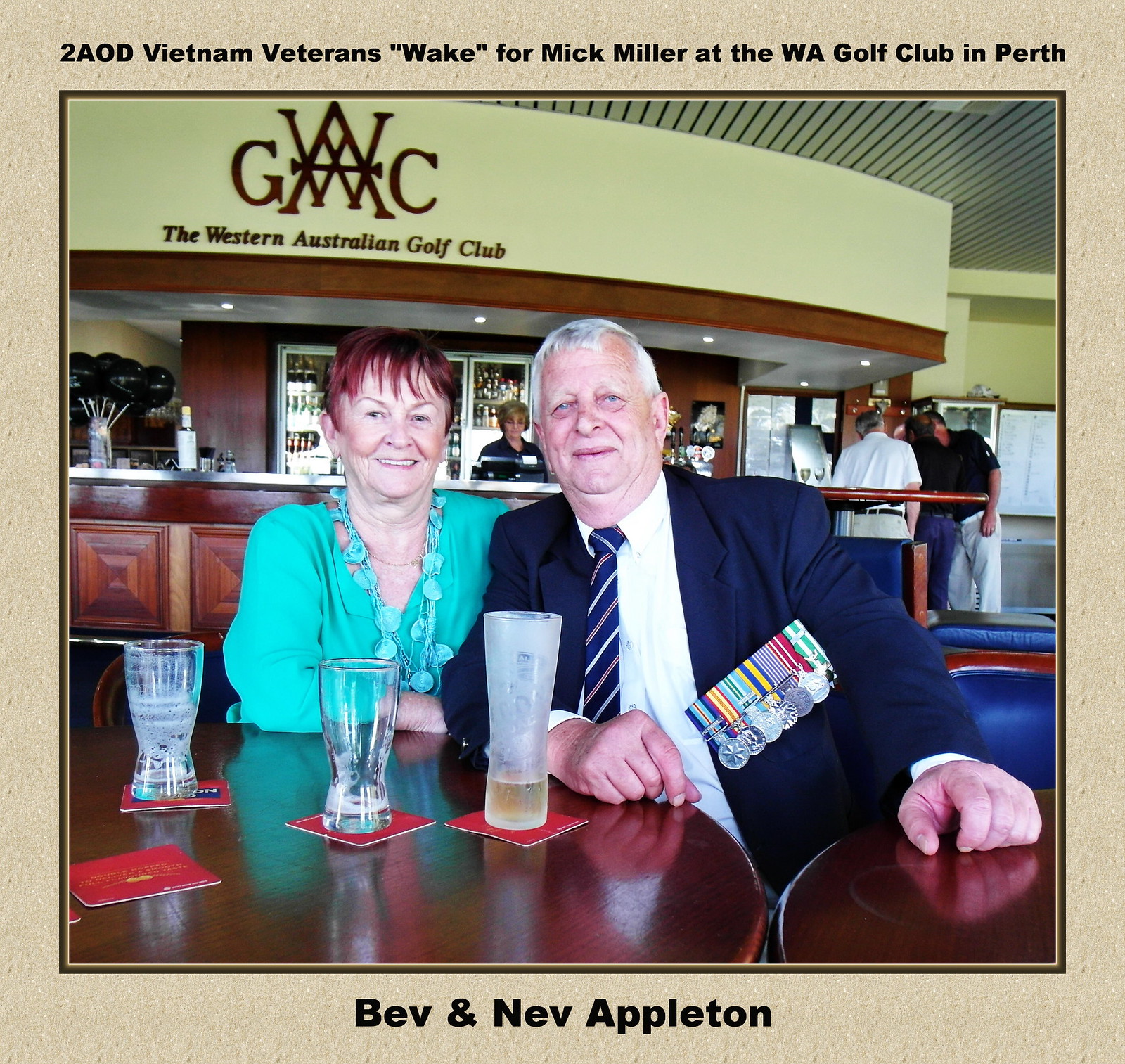In this image, we see a couple, identified as Bev and Nev Appleton, seated at a table inside the Western Australian Golf Club's restaurant area in Perth. A notable part of the setting is the insignia and sign on the wall that likely reads "WAGC" or "WAGWAC," adding a touch of formality to the scene. The man, Nev, is dressed in a blue suit jacket adorned with medals on one chest pocket, a white collared shirt, and a blue tie, while the woman, Bev, wears a green top and has dyed red hair. They appear to be enjoying some beverages, which are visible on the table in front of them. The restaurant features a yellow-painted wall in the background, with multiple people and a server behind a counter, adding to the lively ambiance. The photograph is bordered with a black text caption that reads: "2AOD Vietnam Veterans Wake for Mick Miller at the WA Golf Club in Perth," emphasizing the solemnity of the event.